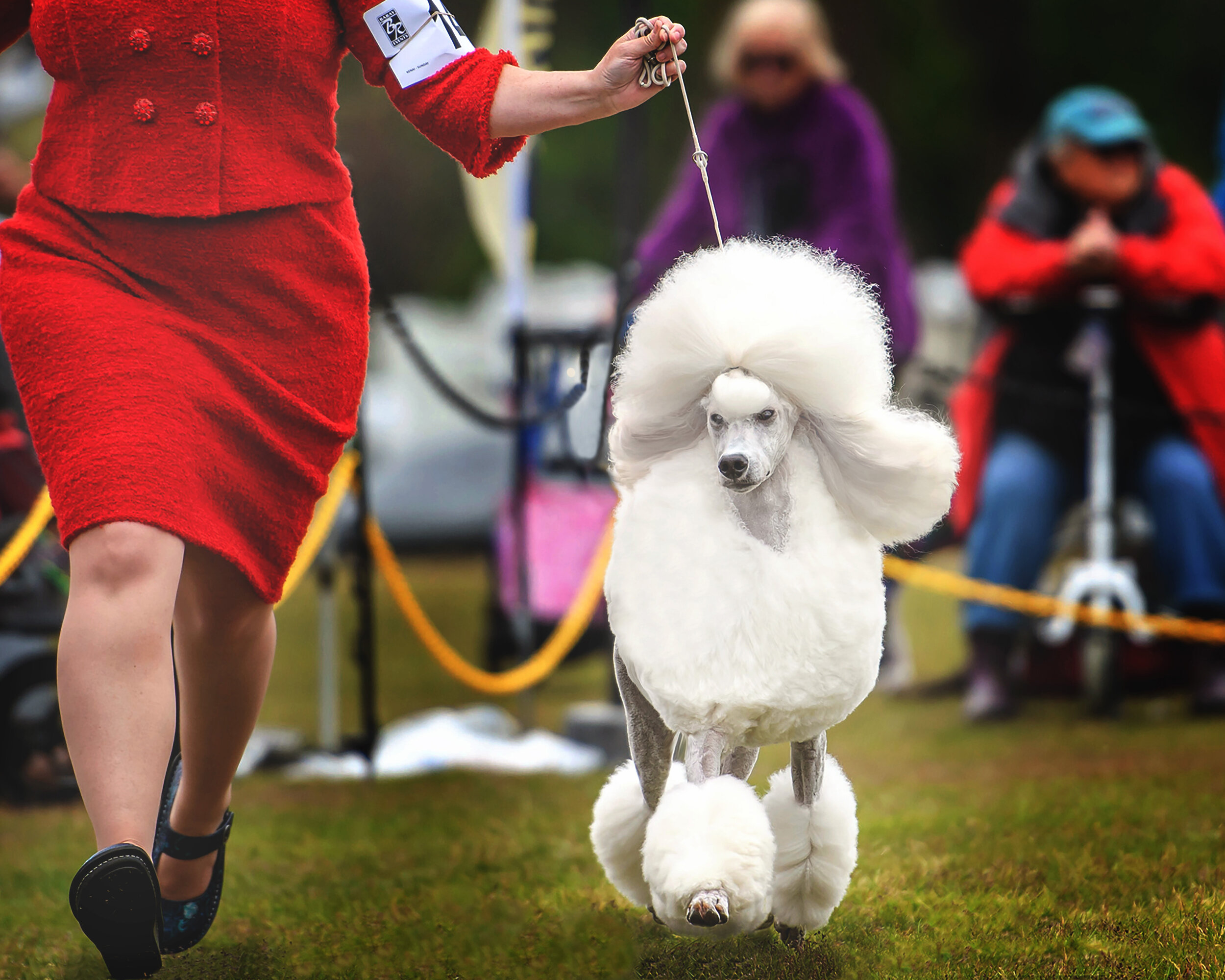In this realistic photograph, oriented horizontally, the setting is a dog show. The image captures a well-groomed white poodle on a short leash, walking across grass. The poodle is in the center of the frame, exhibiting a fluffy body with shaved legs and poofy white hair around the lower legs and head, while its face is neatly shaved. The poodle is being led by a woman dressed in a red boucle dress suit with four buttons on the front, a skirt reaching her knee, and black Mary Jane flat shoes, visible from her shoulders down. She holds a piece of paper in her left hand, potentially related to the contest. In the blurred background, a dark greenish hue suggests trees, with two indistinct figures: a woman in a purple outfit and a man in a red jacket, jeans, and a blue hat, possibly on a scooter. Yellow and black event ropes separate the main scene from the spectators.